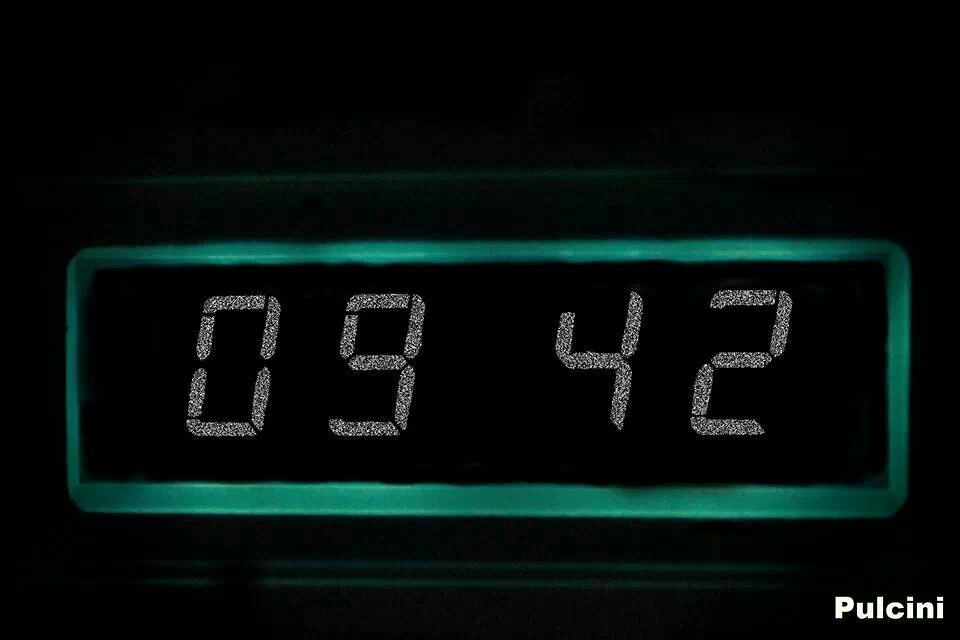A nighttime scene showcases the illuminated face of a digital clock against a completely dark background, emphasizing the clock's soft glow. The landscape-oriented photo features a rectangular outline, faintly visible, framing the clock. This rectangular border emits a gentle, light aqua green illumination, resembling glow-in-the-dark plastic. The clock face itself is an opaque black, contrasting sharply with the silver, glittery digital numbers "09 42" displayed prominently without a colon. In the lower right corner, the word "Pulcini" appears in white, possibly denoting a screen name or watermark.